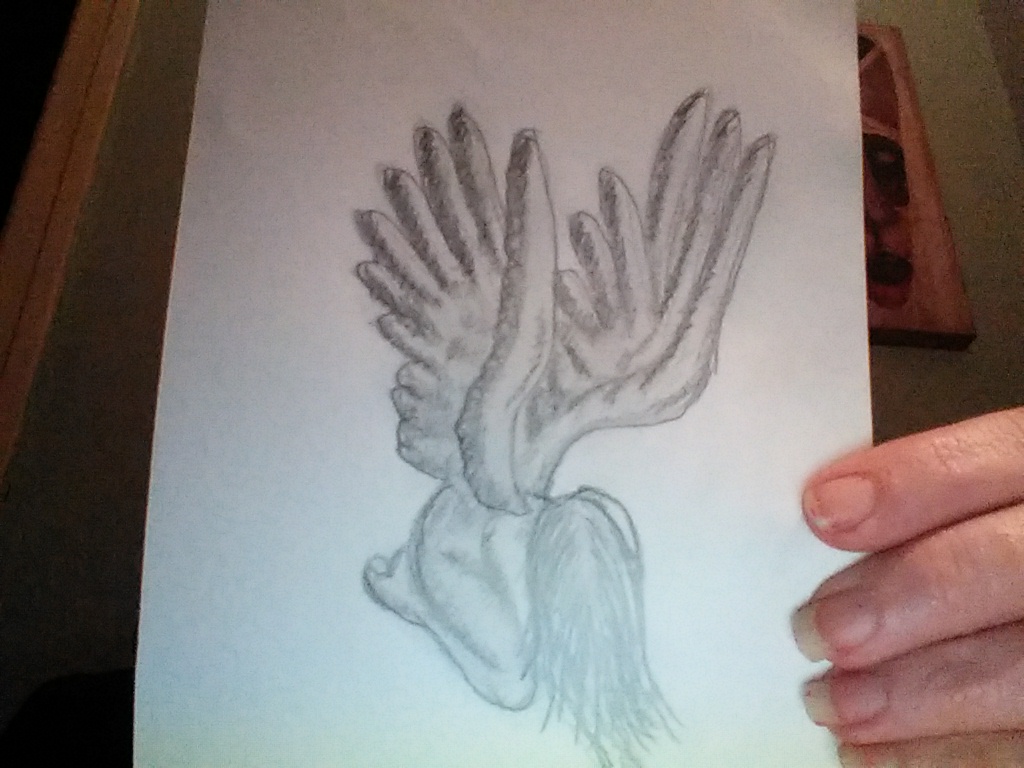The image is a vibrant, color photograph capturing a white piece of paper with a central pencil sketch, held by a woman's hand with long, manicured nails. The sketch features a woman leaning forward, her hair cascading over her face, and her body positioned on her knee with her foot visible. Large wings extend from her back, and the drawing is shaded to emphasize the contours and depth, particularly around the sides of the wings. The sketch is simple and not highly detailed but effectively conveys the posture and ethereal quality of the subject. In the background, there is a glimpse of the woman's living space, visible through the presence of a table on which the paper rests. To the right of the paper stands a wooden object adorned with either a photograph or painting of a mask, adding a touch of artistic ambiance to the scene.